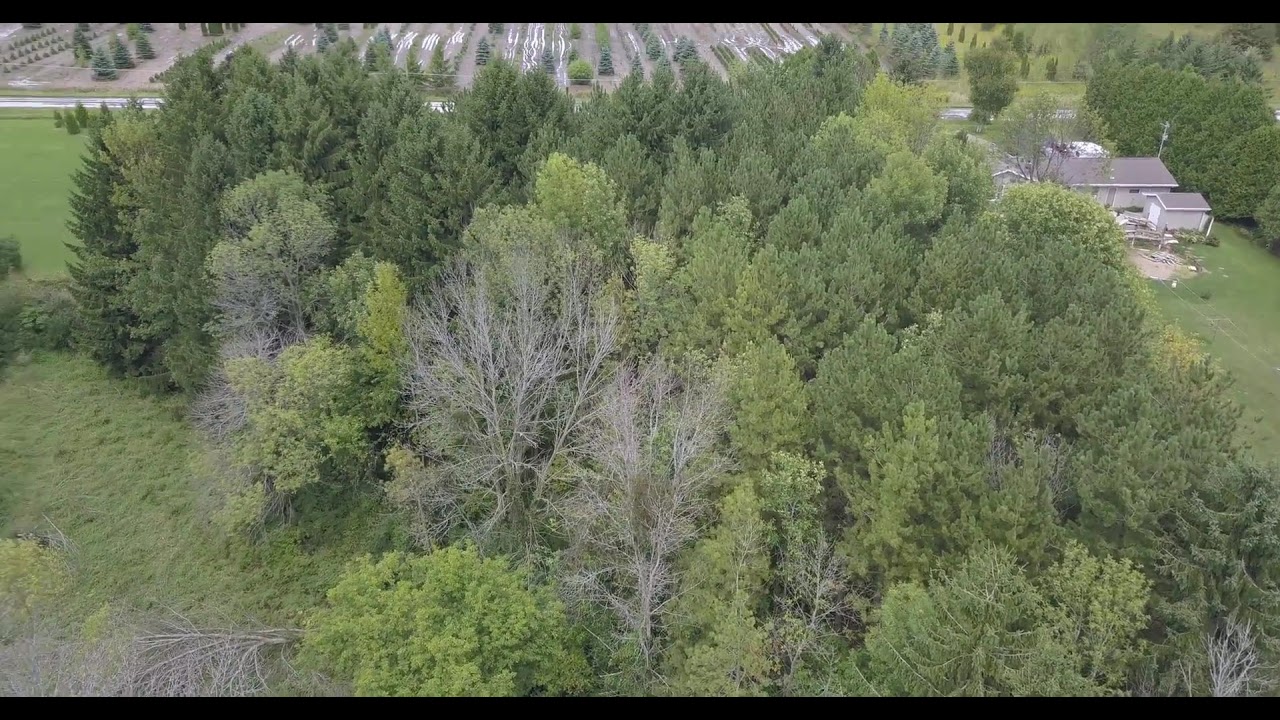This detailed aerial photograph, likely taken by a drone, features a dense and abundant thicket of bushes and trees dominating the center of the image, with varying shades of green foliage. Among the trees, two notable ones on the left are leafless, adding a stark contrast. The left side of the image slopes down onto a hill where a gray fallen tree lies near an open grassy patch. To the upper right corner, a gray house with a dark gray shingle roof partially emerges from behind the trees, fronted by a smaller building with the same siding and roof, including a white door. Adjacent to this is a line of pine trees. In the distance, the image reveals what appears to be rows of crops, difficult to discern clearly, contributing to the agricultural aspect of the scene. Additionally, a narrow gray path runs horizontally across the top left, disappearing behind the dense foliage. The photograph is in color, with a black strip across the top and bottom edges, enhancing the landscape's rich detail and realism, characteristic of drone photography.